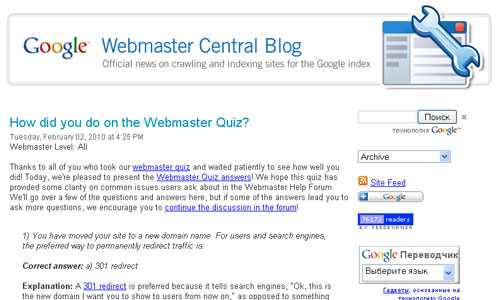The image features a clean, all-white background. At the top, there's a gray-bordered rectangle. On the left side of the rectangle, "Google" is displayed in large letters using its classic colors. To the right of "Google," the words "Webmaster Central Blog" are prominently written in blue. Below that, in smaller black text, it reads, "Official news on crawling and indexing sites for Google Index." 

On the right end of the rectangle, there is a graphic resembling a newspaper outline with a silver wrench overlapping it. Below this section, on the left side, there's a title in vibrant teal blue that reads, "How did you do on the webmaster quiz?" Followed by a question mark. Underneath the title, a date is mentioned, below which it states, "Webmaster Level All."

The main body of text consists of a paragraph of detailed information. Further down, there is a section labeled "1," followed by two lines of text. Below that, it says, "Correct Answer," with information beside it. In bold black text, the word "Explanation" appears, followed by two lines of additional details.

On the right side, there is a search bar. Directly below it, partially obscured text likely reads "Google." Underneath this section, there's another search bar with the word "Archive" in black text. Below, an orange square with a Wi-Fi emblem is visible, accompanied by the underlined text "Site Feed" in blue. 

Further down, there is a gray search bar containing the word "Google." To its right, the tip of the bar is blue featuring a white plus sign. A blue bar below contains a sequence of numbers and letters. At the very bottom, there's a rectangle with "Google" written along with some text in a foreign language, and finally, a search bar with more foreign language text within it.